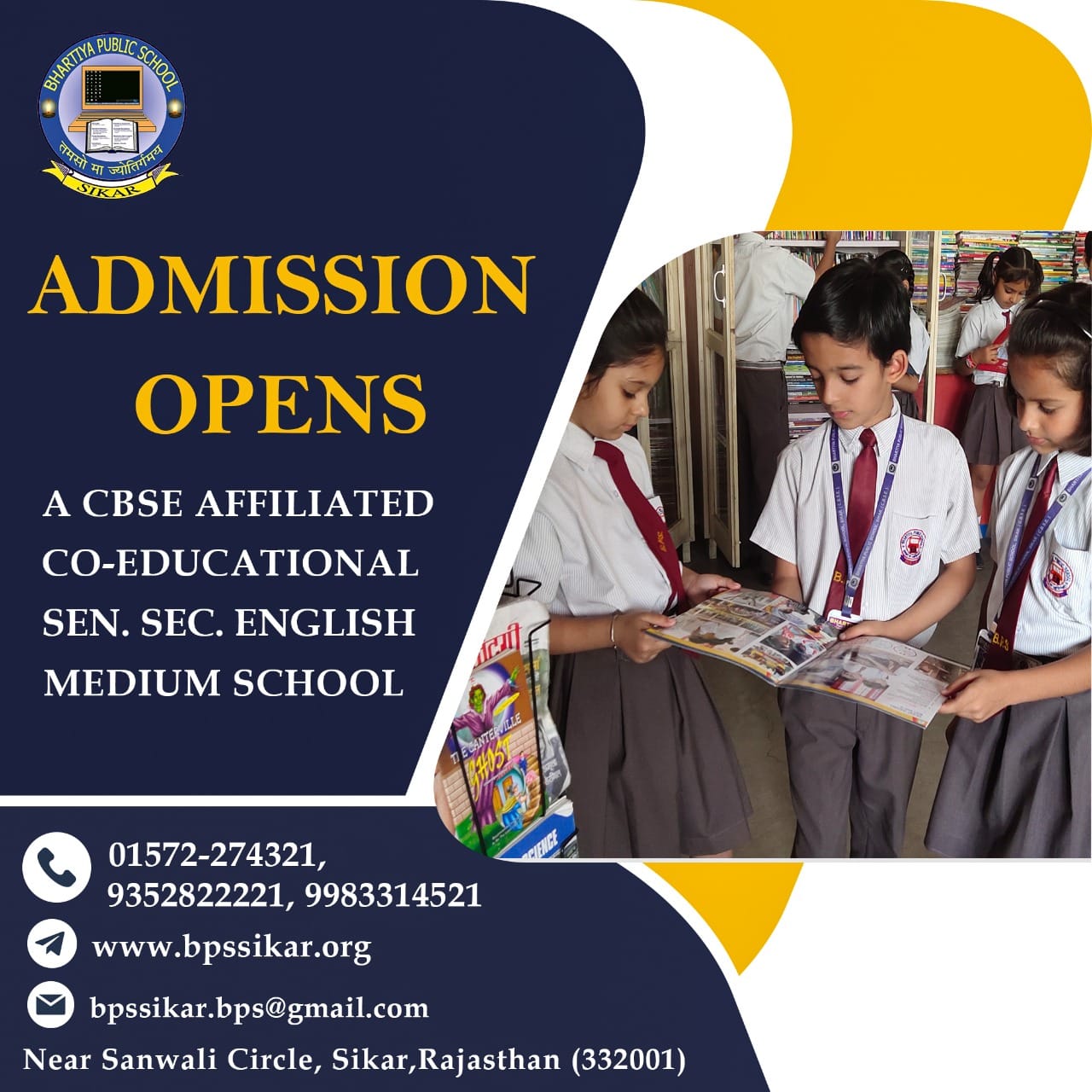The homepage of the Bharatiya Public School website features a prominent image in the upper left-hand corner showing an illustration of a computer with an open book in front of it. Below this image, a small banner reads "SIKAR." The website proudly states that the school is a CBSE-affiliated, co-educational, senior secondary, English-medium institution.

One featured image on the website depicts three children in school uniforms. The uniform consists of buttoned-down shirts with maroon ties, with the boy wearing tan pants and the two girls wearing tan pleated skirts. The boy and the girl on his right are wearing lanyards with identification passes, while the girl on his left has a bracelet on her right hand. All three children are engrossed in a book, sharing it together. In the background, more children are present; some are browsing a bookshelf, and one child is reading in front of another bookshelf. Adjacent to the trio, a bookshelf is visible, with a magazine prominently placed on its side. The page also provides the school's contact number, website address, and location details.